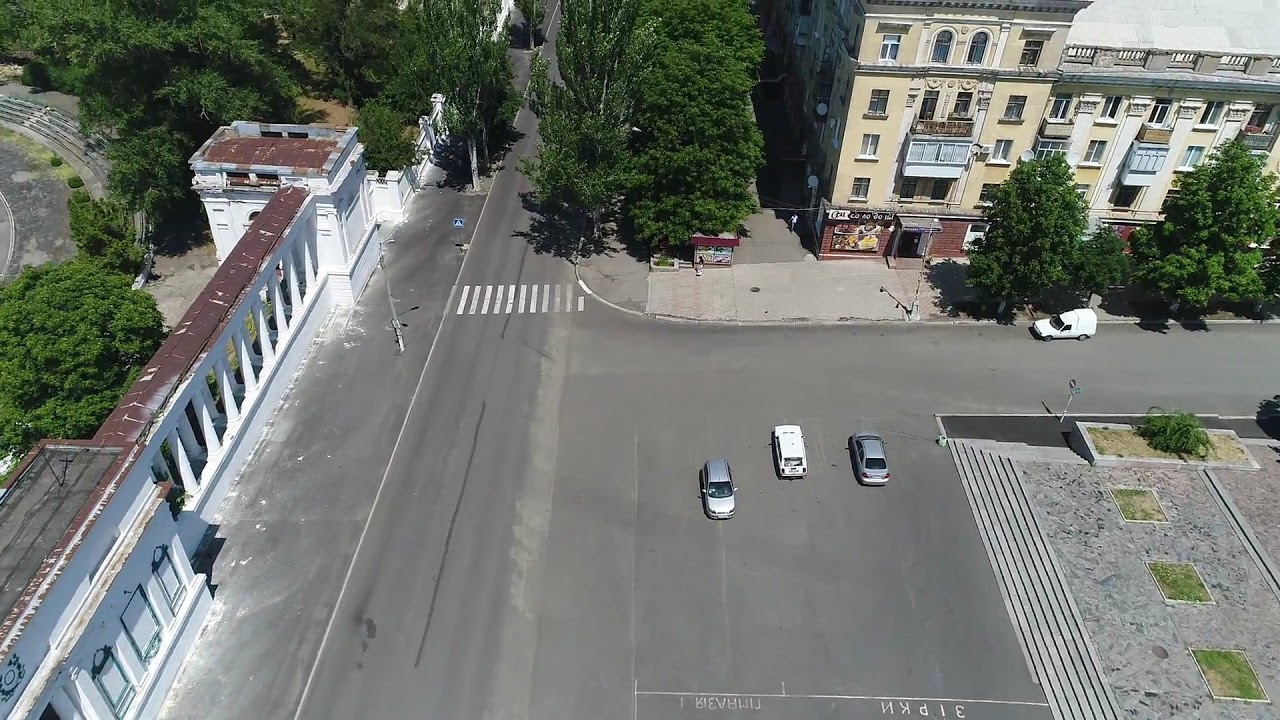This aerial image captures a bustling urban scene. In the center, there's a large parking lot with three cars scattered across it, although the parking area isn't visibly lined, giving it an unusual appearance. Adjacent to the lot is a wide road running from the front to the back of the frame, featuring a pedestrian crossing that connects to a sidewalk. 

On the right-hand side, there is an old apartment building with five floors at one section, mainly yellow with a brown brick base. The building's center is white, highlighted by a lone balcony and a storefront at the bottom displaying a food sign. This structure is attached to a four-story building adorned with white pillars and similar yellow coloring. The area in front of these buildings is lined with trees and features a small park area with gravel paths and steps, providing a modest green space amidst the urban environment.

To the left of this urban center, there is a long wall of white pillars connecting two structures, creating a frame for the scene. Below this, a road runs parallel bordered by trees, leading to another zone with white, shop-like buildings along a sidewalk. The overall setting merges residential and commercial elements, indicative of a lively neighborhood where people live, shop, and traverse daily.